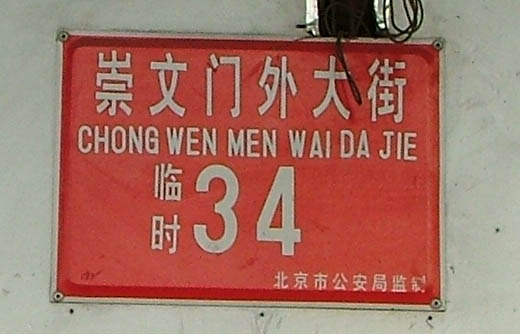This landscape-oriented photograph captures a street sign mounted on an off-white concrete wall, displaying imperfections such as lighter grey patches and black spots. The sign, set against a backdrop of smooth but blemished concrete, features traditional Japanese characters at the top, followed by pinyin transliterations: "CHONG, WEN, MEN, Y, W-A-I, DA, G, J-I-E." Below these transliterations, the number 34 is prominently displayed. The sign itself is a striking red with a thin silver or light beige border and an even finer outermost white line. Suspended above the sign, an enigmatic object with an aluminum side and a black center has wires extending from it into the wall, potentially powering a light for the sign.